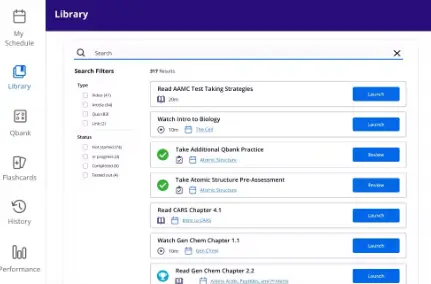This screen capture showcases the interface of an educational platform, characterized by a variety of icons and tools for user navigation and interaction.

On the left side of the image, there is a vertical, white toolbar featuring a series of icons primarily in gray, with one in blue. From top to bottom, the first icon is a calendar labeled "My Schedule." Following this is a blue icon labeled "Library," illustrated with an open book and a blue bookmark. The next icon, although slightly blurry, appears to say "Q Bank" and depicts a paper with various symbols on it. Below it is an icon for "Flashcards," represented by a set of flashcard symbols. Further down, "History" is identified with a clock and an arrow icon. Finally, an icon for "Performance" features a bar graph.

To the right of the toolbar, a prominent royal purple bar with white text reads "Library." Below this bar, there is a white search box with a gray magnifying glass icon and the word "Search" in gray text. A thin blue line underlines the search box, and a gray "X" is visible within it, likely for clearing the search input. Adjacent to the search box are search filters, labeled "Search Filters" in black. These filters are divided into categories, each with boxes containing text that is too small to decipher.

Beneath the filters and search box, seven white, gray-outlined boxes are displayed. Each box contains various icons and black text, including blue boxes with white text indicating actions like "Watch Intro to Biology" and practice activities. Some boxes feature green circles with white check marks, signifying completed tasks or achievements. Above the first gray and white box, the number of search results is displayed.

Overall, the image effectively highlights different sections and functionalities offered by the platform, aiding in user navigation and resource management.